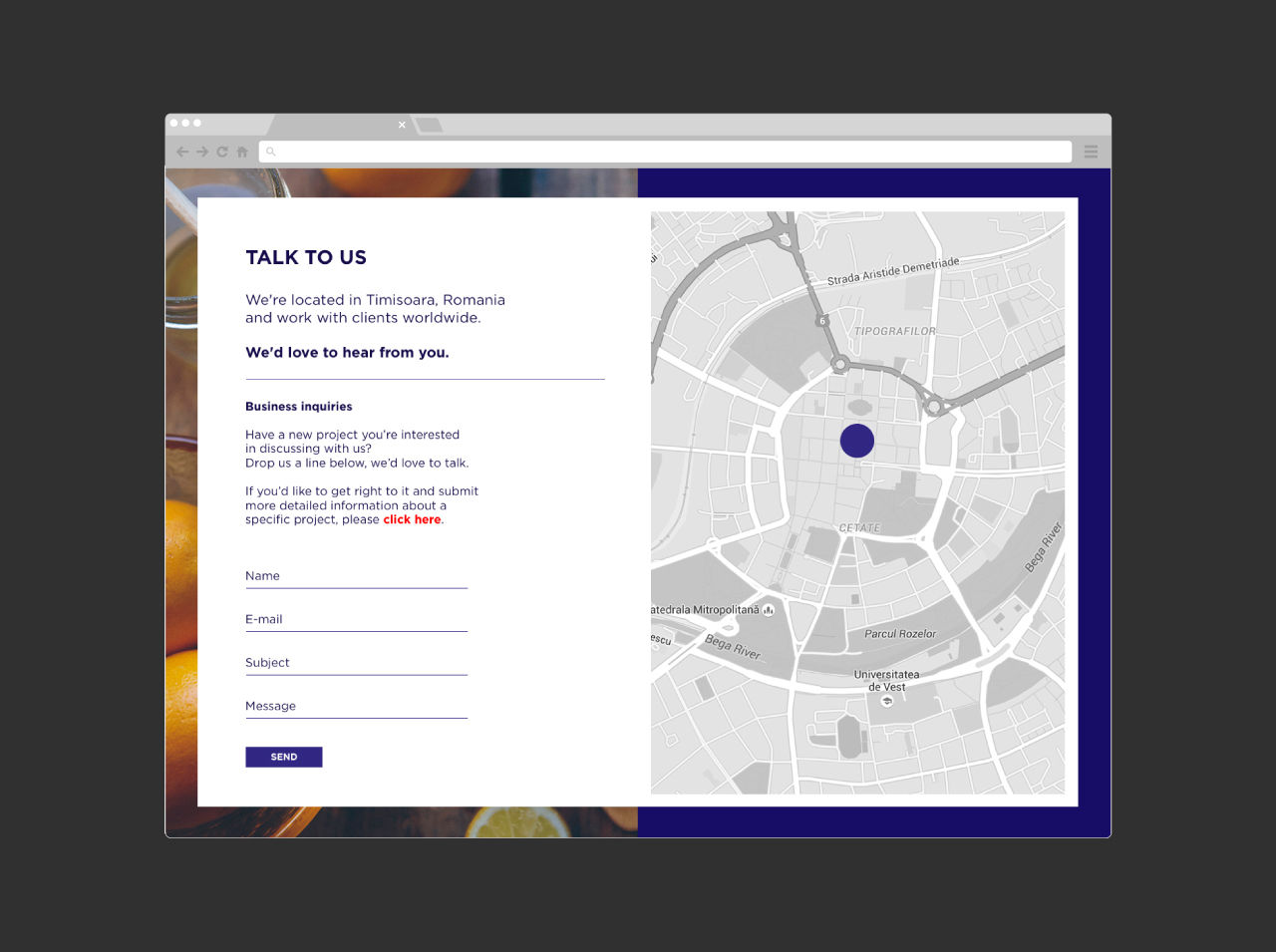This image showcases a webpage with a dual-colored background split into two sections. The left side features a close-up of sliced oranges, set against a backdrop that transitions from dark gray to nearly black. The vibrant oranges add a pop of color and suggest a culinary theme. On the right side, there is a royal blue, almost navy blue area that is overlayed with a transparent rectangle containing a map.

The map has a blue dot towards the center, indicating a specific location. Above the map, there are text sections inviting user interaction. The text reads: "Talk to us. We're located in Timișoara, Romania, and work with clients worldwide. We'd love to hear from you." It further prompts business inquiries with the message: "Have a new project you're interested in discussing with us? Drop us a line below. We'd love to talk." Another line encourages users to click for more detailed project information, with "click here" highlighted in red.

Below this text, there is a form with labeled lines for user input, including fields for "Name," "Email," "Subject," and "Message." At the bottom of the form, there is a blue rectangle button with the word "SEND" in all capital white letters, inviting users to submit their details. The overall design combines professional and vibrant elements to engage the viewer effectively.